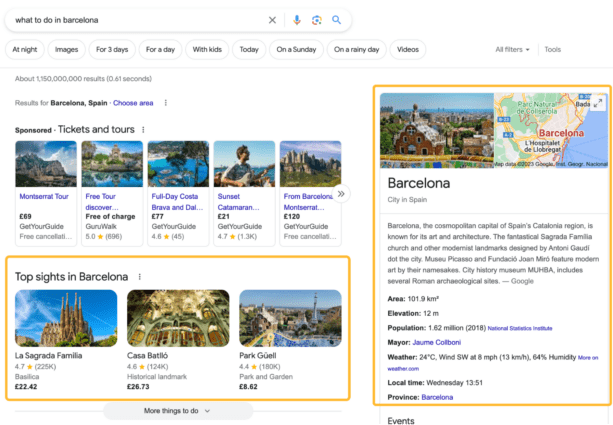A detailed and cleaned-up caption for the given image description:

"A Google search results page screenshot with the query 'what to do in Barcelona' displayed in the search bar. The upper left corner features Google's logo, while the search bar includes icons for Voice Search (microphone), Camera Search, and the traditional search button. Below the search bar, there are various filter options displayed as clickable buttons, which include 'at night,' 'images,' 'for three days,' 'for a day,' 'with kids,' 'today,' 'on a Sunday,' 'on a rainy day,' and 'videos.' On the right side of these options are links for 'All filters' and 'Tools.'

The search results show approximately 1.15 billion results generated in 0.6 seconds. The top results from 'washable stripping' (likely a misinterpretation) include different areas of Barcelona, featuring tickets, tours, and hotels. Below this listing, a yellow-highlighted section titled 'Top Sites in Barcelona' features an image of the Sagrada Familia, the iconic church perpetually under construction, and other notable landmarks in Barcelona. There are also options for park tours and pricing information.

To the right of the main search results is a detailed informational panel about Barcelona, including a map of the city. The panel provides a brief description: 'Barcelona, a city in Spain,' followed by specific details about the city such as its area in square kilometers, elevation, population, current weather, local time, the province, and the name of the current mayor."